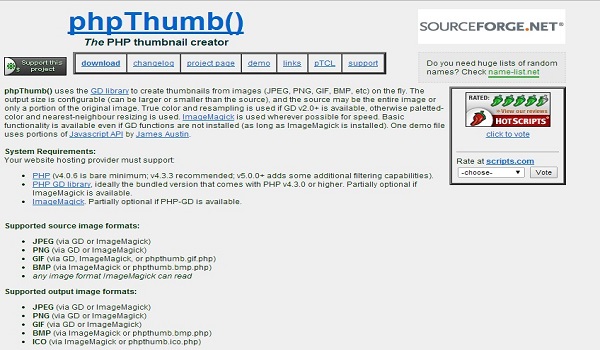The image showcases a section of a website detailing the features of "phpThumb". At the top, the header reads "phpThumb, the PHP Thumbnail Creator". Below the header, a description explains that phpThumb utilizes the GD library to generate thumbnails from various image formats such as JPEG, PNG, and GIF in real-time. The output size of these thumbnails is configurable, allowing for dimensions larger or smaller than the source image. Additionally, the source can be either the entire image or just a portion of it. 

For high-quality rendering, true color and resampling are used if GD v2.0 or later is available; otherwise, paletted color and nearest-neighbor resizing are employed. Wherever possible, ImageMagick is utilized to enhance processing speed. Even if GD functions are not installed, basic functionality remains accessible provided that ImageMagick is available. The image also mentions that one of the demo files integrates portions of a JavaScript API developed by James Austin.